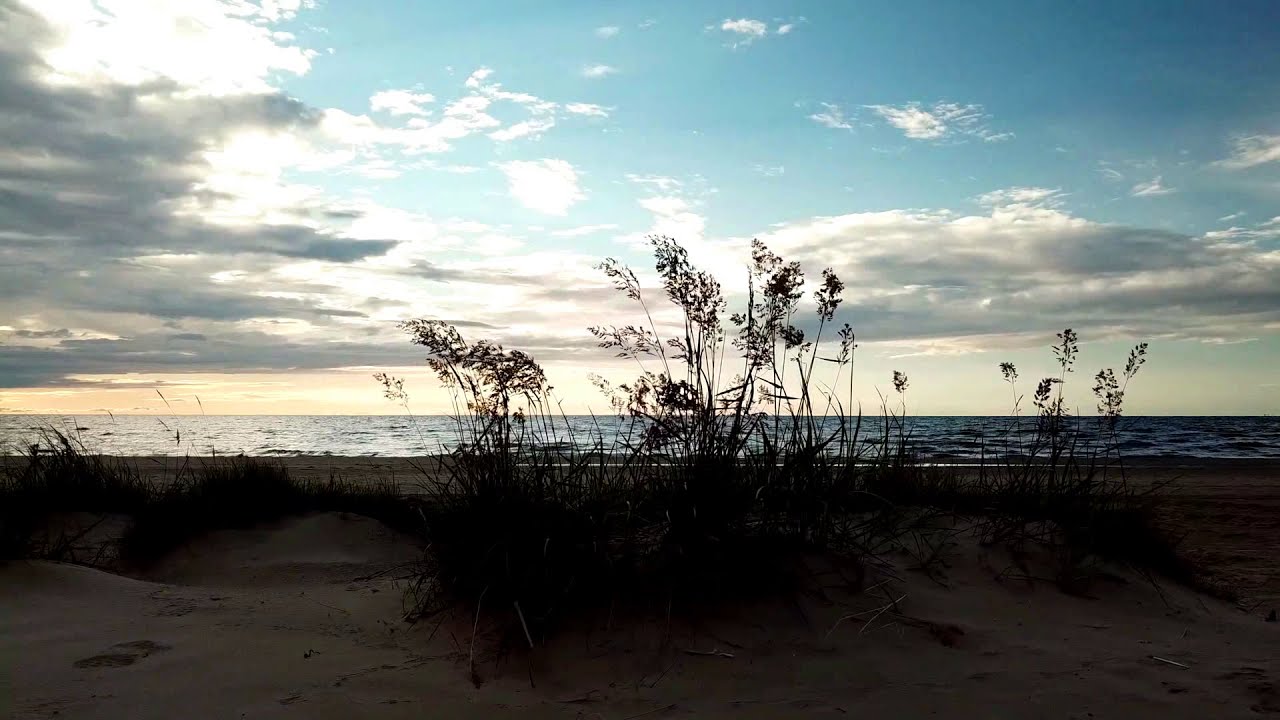This photograph captures a serene beach scene at dusk, just before sunset. In the foreground, sand stretches across the bottom third of the image, adorned with dark silhouetted plants and weeds whose tops reveal some indistinct leaves. The middle portion features a vast, calm expanse of blue ocean or lake, extending from left to right. The horizon splits the image, with the expansive sky occupying the top half. The sky is a patchwork of blue, white, and gray clouds, with some dramatic lighting created by the sun obscured behind the clouds. The overall hue and light indicate the impending sunset, casting a tranquil ambiance over the scene. The entire photograph is devoid of people or text, focusing purely on the natural beauty of the landscape.